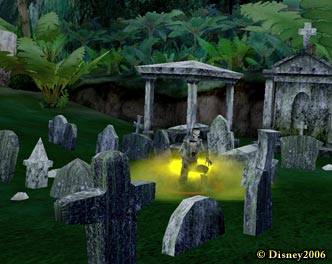In this vibrant, fantasy-style, computer-generated image of a graveyard from a video game, we observe a landscape filled with various gravestones. These headstones form a traditional cemetery scene with a lush green grass covering the ground. Central to the composition is a gravestone enveloped by a yellow, gaseous smoke, giving the eerie appearance of a ghostly figure emanating from the luminous haze. Surrounding this spectral center are numerous cross-shaped and conventional headstones. In the top right corner, a mausoleum seems to loom partially veiled by the yellow fog, while a small gazebo can also be discerned within this misty area. The top left corner features a striking palm tree plant rooted in the ground. The entire scene exudes a haunting, yet captivating atmosphere, accentuated by the copyright mark "Disney 2006" in the bottom right-hand corner.